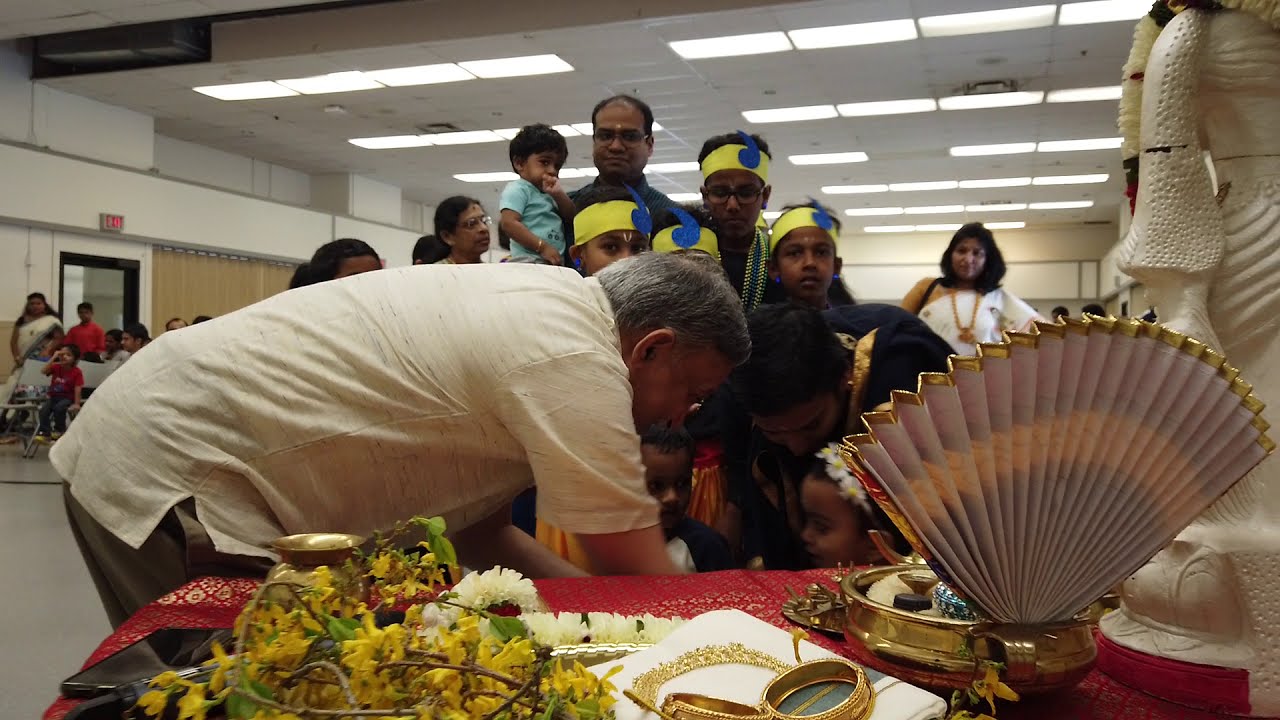In a brightly lit hall adorned with large square fluorescent lights and an exit sign over the doorway, a celebratory gathering is in progress, hinting at a possible Indian wedding or graduation ceremony. Central to the scene, a table is draped in a vibrant red tablecloth, adorned with yellow floral garlands and gold embellishments, including a delicate fan with a gold fringe set in a bronze urn. Among the various items, there are gold bracelets, a book, a phone, and a small white statue, possibly of religious significance.

An older man with greying hair, possibly the patriarch, leans over to interact with two young children at the table, as if instructing or gifting them something significant. Surrounding them, a mix of kids and adults can be seen, including four children with distinctive yellow headbands adorned with blue dots and feather-like decorations. The atmosphere is filled with familial warmth and cultural richness, indicative of a special family celebration or religious ceremony.